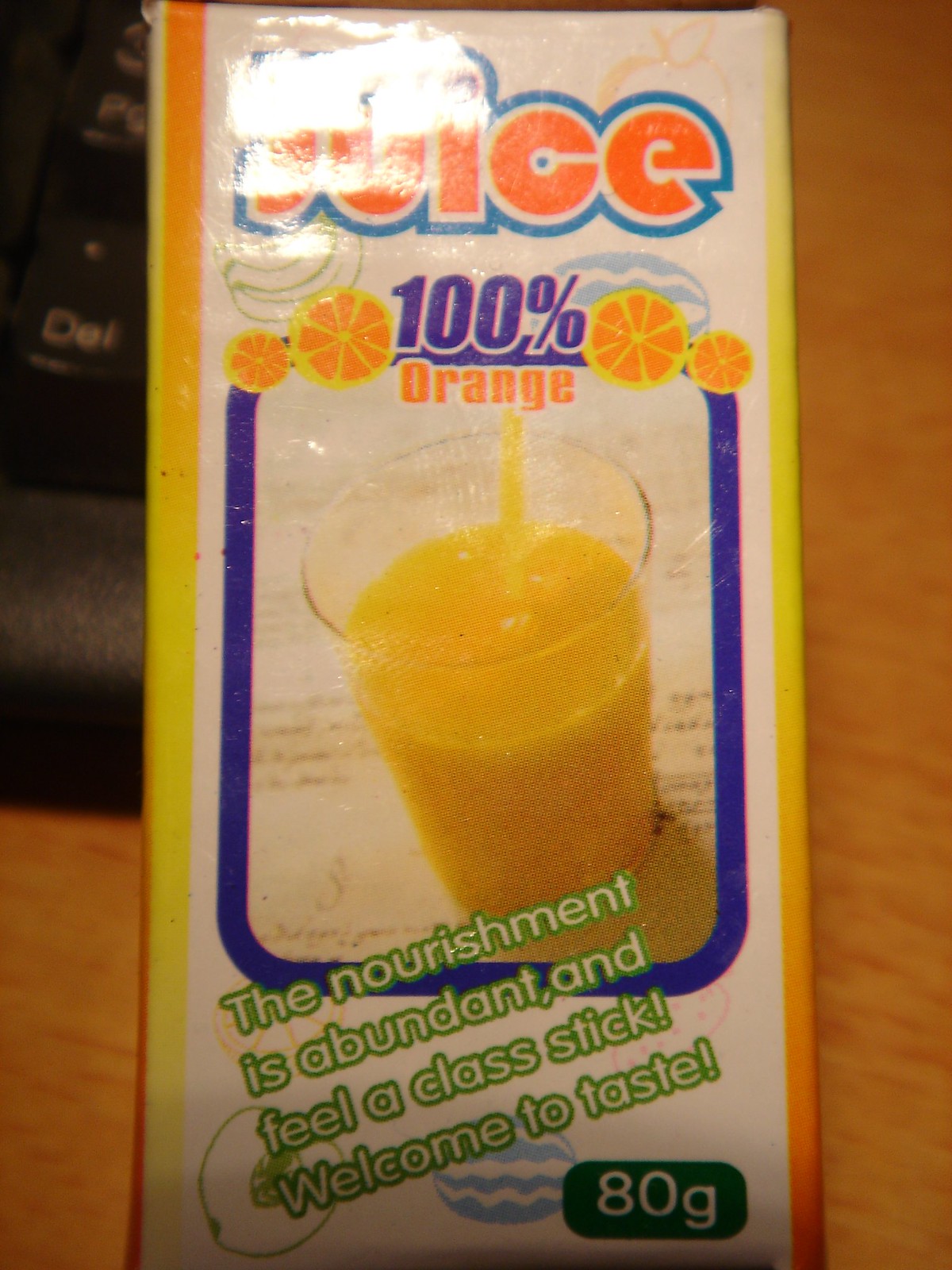Photograph of an orange juice drink in a juice box format. The top of the juice box displays some glare, making it difficult to read the product name, but it appears to say "Juice" in orange letters outlined in blue. The center of the juice box features an image of orange juice being poured into a glass, framed by a purple border. At the top, the juice box prominently declares "100% Orange Juice," accompanied by small images of orange slices. Below the glass image, text in green letters outlined in white reads, "Nourishment is abundant and feel a classic. Welcome to taste." At the lower right corner, the juice box indicates the quantity with "80 grams" in green text.